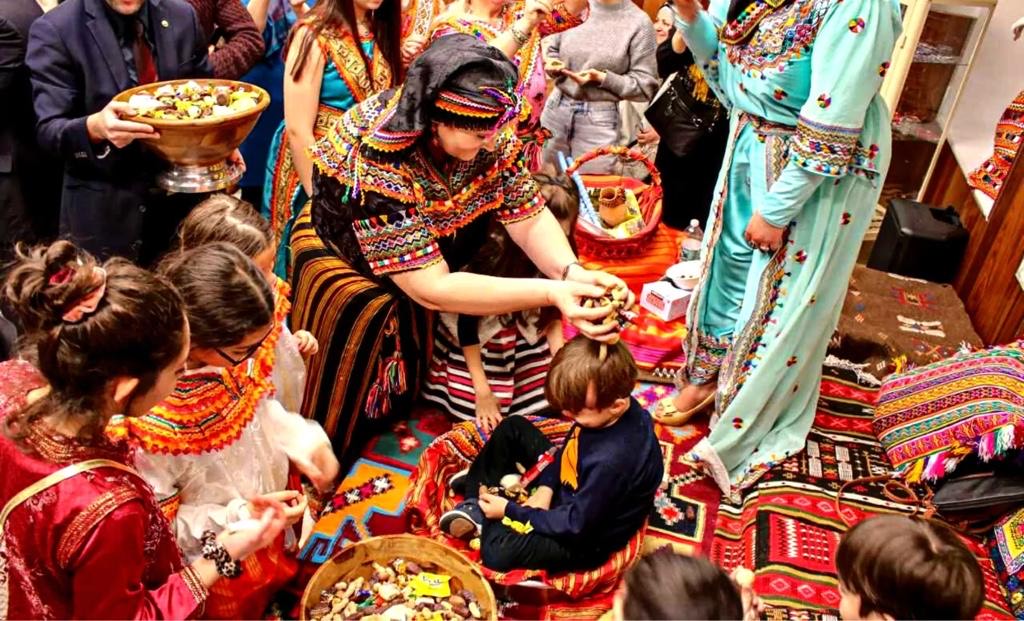This vibrant and lively indoor photograph captures a ceremonial scene, likely from a cultural festival. Dominated by rich tones of red and orange, the image is bustling with detailed patterns and colors, creating an intricate visual tapestry that's both captivating and overwhelming. In the center of the scene, a small boy, dressed in a dark blue outfit with black trousers and blue shoes, sits in a bowl-like basket lined with a reddish-orange blanket. His short brown hair and folded legs highlight his youthfulness, estimated to be around five years old.

To the boy's right, an older woman in a highly embroidered black dress with yellow, orange, green, and white accents, and a distinctive black headdress adorned with yellow, orange, and black stripes, is seen sprinkling what appears to be nuts, grains, or candy over his head. Her hands are raised in an anointing gesture, emphasizing the ceremonial nature of the act. Some of these items have landed in the boy’s lap as he looks down.

On the stage, beside the boy, stands a woman in a long, turquoise gown decorated with several medallions, adding to the colorful contrast of the scene. In the foreground, another woman in a colorful outfit holds a bowl filled with similar nuts and grains, hinting at their significance in the event.

The setting suggests a small stage with people gathered around, including three girls standing to the left, dressed in red and white dresses, and two boys with short brown hair in the bottom right corner, partially visible. A gentleman in a dark suit can be spotted in the upper left corner, partially cut off, holding a similar bowl of organic-looking elements. The scene is intricately adorned with colorful carpeting and blankets, potentially muddling the exact cultural origin but suggesting influences possibly from the Indian subcontinent, Central or South America, Persia, or Afghanistan, given the exotic and elaborate designs.

Overall, this photograph beautifully encapsulates the essence of a cultural ceremony with a rich, multicultural aesthetic, displaying anointing rituals amidst a kaleidoscope of vibrant colors and textures.